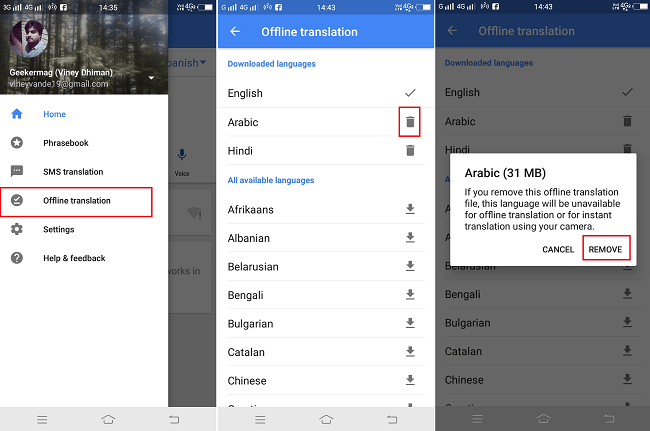The image showcases a composite of three smartphone screens aligned side-by-side, providing a comprehensive view of various features and settings within an application. 

On the far left screen, the user's profile is prominently displayed. It includes the name "Geekermag Vinnie Demmon" accompanied by an email address. At the top, there's a circular avatar featuring a man's photo set against a backdrop of forest trees. Below this, several icons and labels are listed vertically, starting with a blue icon labeled "Home," followed by a white star in a circle tagged as "Phrasebook." Next is a speech bubble with dots titled "SMS Translation," a check mark over a book labeled "Offline Translation," a gear icon for "Settings," and finally, a question mark icon labeled "Help and Feedback." Notably, the "Offline Translation" section is highlighted with a red rectangle, drawing attention to this feature.

The middle screen focuses on language settings, specifically Arabic. Here, the user appears to be in the process of selecting a trash can icon adjacent to the Arabic language option. 

On the farthest screen to the right, a prompt is visible, warning the user about the consequences of removing the Arabic offline translation file. The message reads: "If you remove this offline translation file, this language will be unavailable for offline translation or for instant translation using your camera." The option to remove the file is accentuated with a red rectangle surrounding the word "Remove."